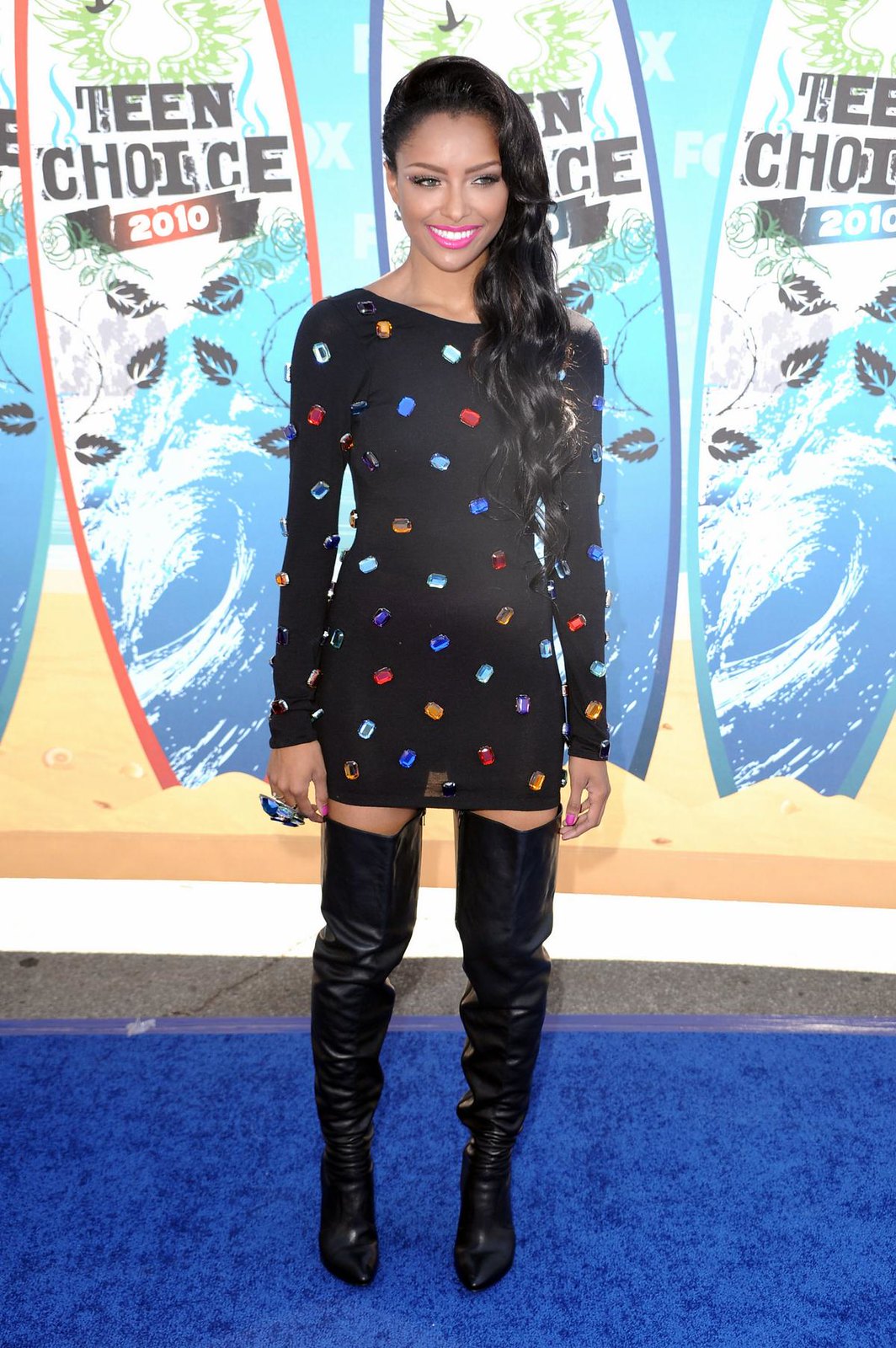This image captures an African-American woman standing confidently at a press event in front of a backdrop adorned with three surfboards, each inscribed with "Teen Choice 2010." The surfboards feature vibrant outlines in orange, blue, and turquoise, accompanied by designs of waves to evoke a beach theme. The woman, who appears to be in her late teens or early 20s, has long dark hair swept elegantly over her left shoulder. She is beaming with a smile and is dressed in an eye-catching black mini dress. This dress, characterized by its long sleeves and short hemline, is decorated with colorful, inch-wide faux gemstones dispersed in a sporadic pattern, creating a playful polka dot effect with hues of red, blue, yellow, and clear. Complementing her outfit are black ruched leather boots that extend above her thighs. Standing on a blue shag carpet, the woman looks slightly to the right with both arms relaxed at her sides, set against an asphalt surface beneath the vibrant backdrop, signifying her arrival at the Teen Choice Awards.